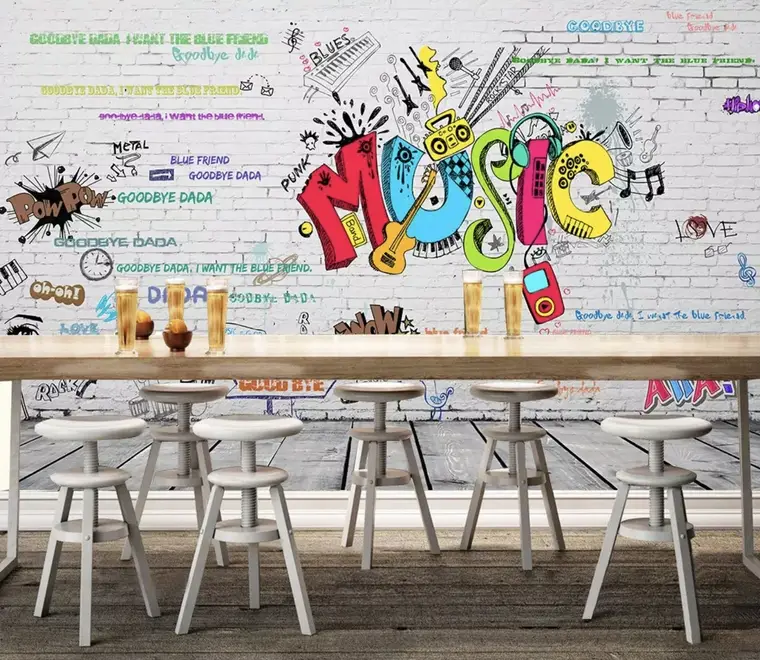This photograph captures a digitally-created, vibrant scene set in what appears to be a lively cafe. The centerpiece of the image is a long, light brown wooden table with sturdy white tripod legs, surrounded by adjustable white barstools with screw-like seats. Arrayed on the table are several tall, clear glasses filled with a golden liquid, possibly beer, topped with white froth, alongside a couple of small brown bowls containing oranges.

Dominating the backdrop is a bright white brick wall adorned with an eclectic and colorful mural. The word "MUSIC" is prominently displayed in large, artistic letters in varied hues—red M, blue U, green S, pink I, and yellow C. The mural ingeniously incorporates musical imagery: a guitar stretches across the M and U, piano keys are depicted below the U and across the C, a yellow boombox is positioned above the U, and a pair of green headphones dangles from the I, connected to an iPod.

Additional graffiti, including comic book-style words like "Pow Pow," signatures, hearts, and phrases such as "Goodbye" and "Goodbye Dada," are scattered around the mural. Music notes, horns, and other doodles in vibrant colors—red, blue, orange, green, pink, teal—further embellish the wall, adding to the lively and whimsical atmosphere of the scene. The overall ambiance suggests a fun and inviting place to visit.